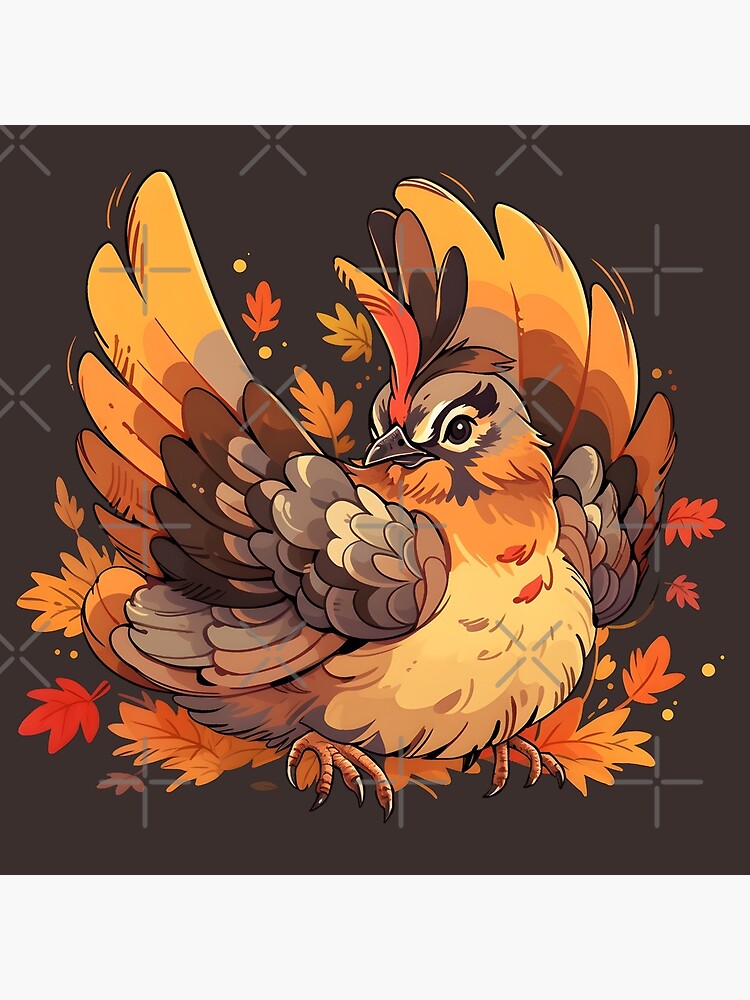This digital illustration features a charming cartoon turkey positioned against a dark, slightly brownish-gray background adorned with watermark patterns of Xs and plus signs. The turkey exhibits a variety of fall and Thanksgiving colors. Its plumage showcases a gradient from light brown to darker brown to vibrant oranges and yellows. Specific details include a light yellow, rounded stomach, and layers of feathers on its wings, transitioning from brown at the base to bright oranges and reds at the tips. The turkey's head, turned slightly to the side, is a brownish hue with an orange neck, complemented by a sprout of red and brown feathers enduringly perched above its beak and one visible black eye. Positioned at the bottom of the image are red-orange and yellow foliage leaves, imply a seasonal autumn theme, adding to the rich, celebratory ambiance of the artwork. This polished and professional piece emanates warmth and festivity, suitable for Thanksgiving-themed contexts.